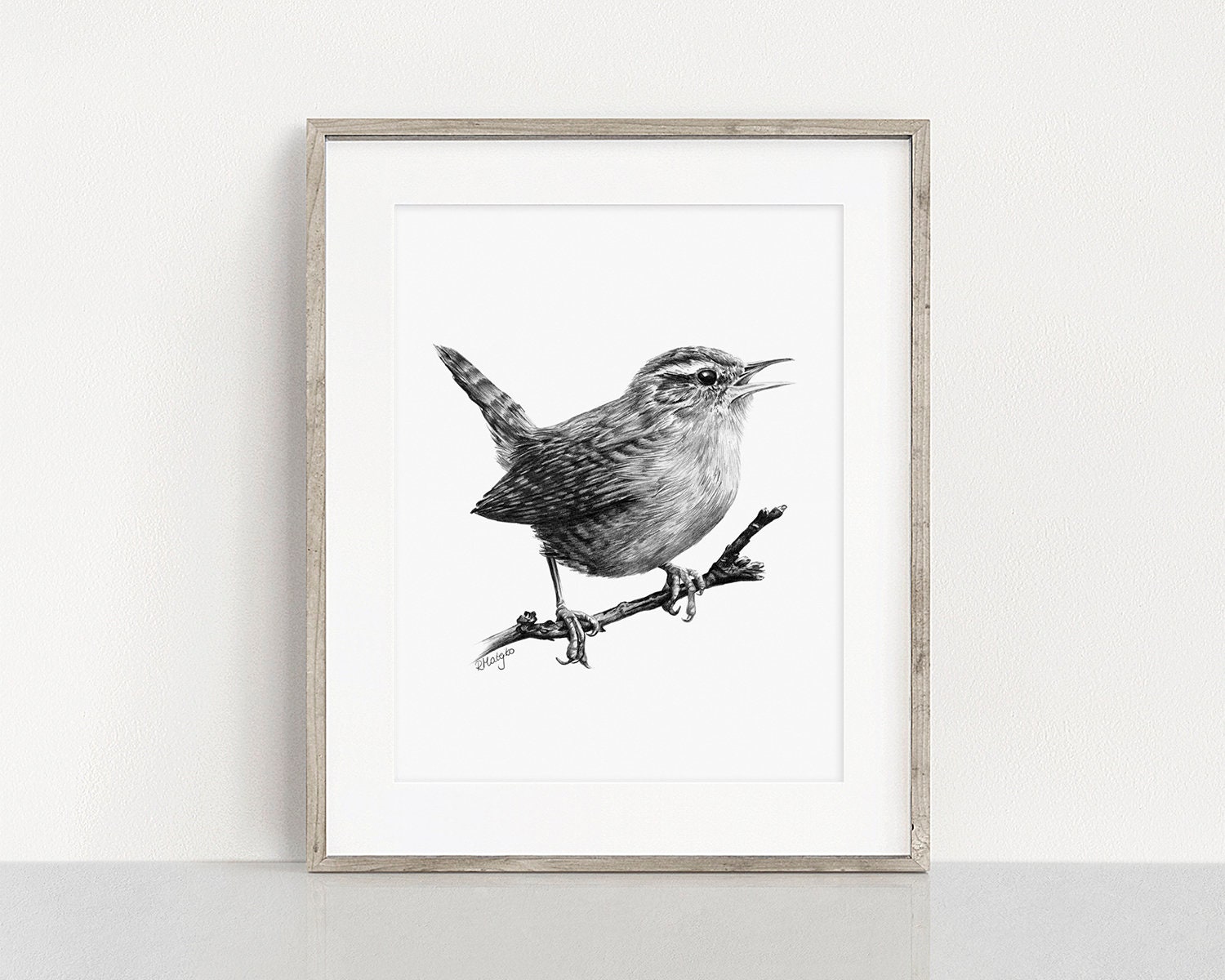The photograph depicts a square framed picture of a detailed black and white drawing or sketch of a European wren perched on a branch. The image is set against a blank white background. The wren, facing to the right with open eyes and an open beak, sits centrally within the frame, which is composed of thin, light gray wooden material. The frame includes a white mat border. The drawing is likely done with pencil or pen and ink and is signed beneath the branch. The photograph itself shows a very even, professional lighting setup, indicating it was taken in a studio. The backdrop of the photo is a very light gray to bluish-gray, almost white, and features a slightly darker gray strip running along the bottom. The image conveys a minimalistic yet meticulously detailed depiction of the small bird, highlighting its compact form, prominent tail, claws gripping the branch, and its alert expression as it seemingly watches for potential prey.